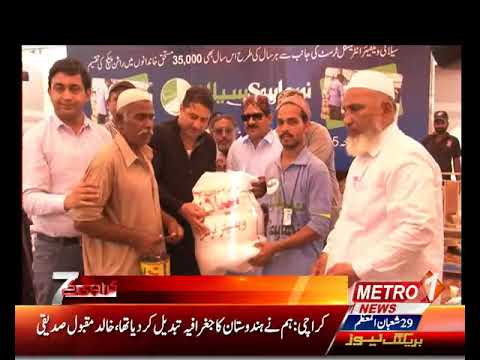This photograph appears to capture an event likely set in an Arabic-speaking region or involving Arabic-speaking people, possibly located in India or Pakistan, as suggested by the presence of both Arabic and Indian languages. The scene showcases a group of approximately eight to ten men standing together in a large room, posing with a substantial white object that resembles a bag or box. The men are dressed variably, including traditional Muslim attire with beards and white caps, casual polo shirts, and button-down shirts. One man, notably, is in an all-white outfit with a matching cap and white beard, while another wears sunglasses. 

In the background, a vibrant blue banner adorned with Arabic script and numbers, including "35,000," adds context to the occasion. The banner may also display charts and photographs. The men are standing behind a wooden table, with a perceived security guard in black uniform visible at the rear. An orange band with white text, which includes "Mentor News" in English, runs along the bottom of the image, typical of a TV news program interface, accompanied by additional banners and text in multiple languages, including Indian scripts. The detailed setup, attire, and diverse script suggest a formal or celebratory gathering, possibly to announce or receive a reward or recognition.